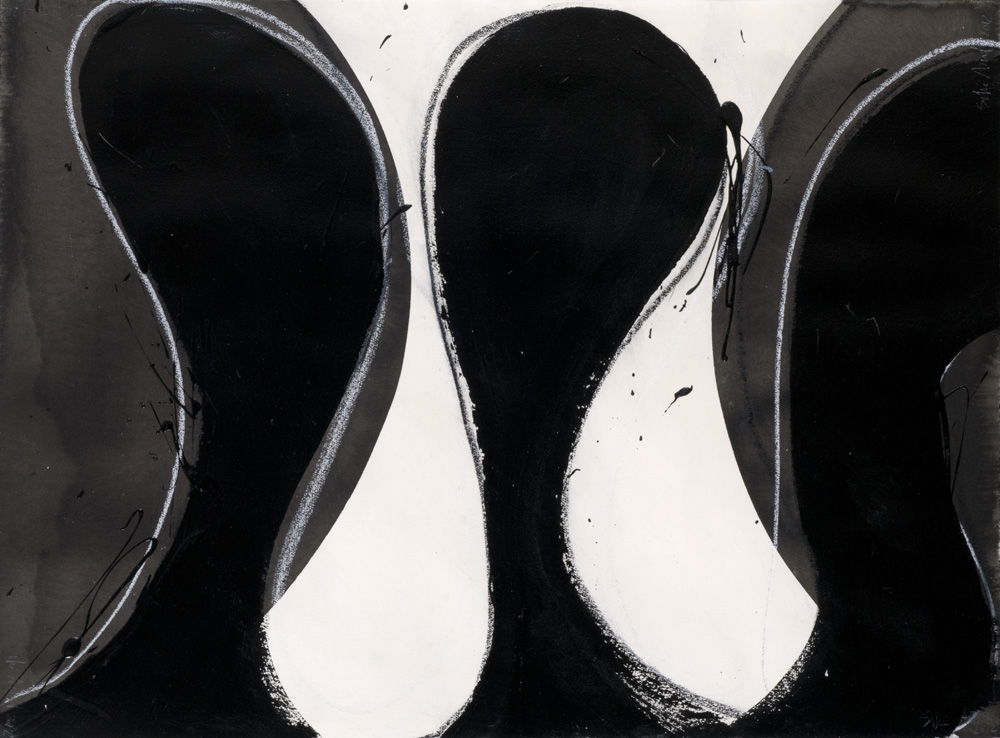This is an abstract black and white painting with hints of blue and cream. The artwork features several rounded and oblong shapes extending upwards from the bottom, reminiscent of bodies with elongated necks and oddly shaped heads. These shapes appear almost like inverted water drops, predominantly in black and outlined in white chalk, against a white and gray background. The painting also incorporates wavy, lava lamp-like figures that evoke the flow of ink or slime, creating a dynamic movement throughout the canvas. Notably, a large, roundish figure on the right side has a blue ribbon-like element that extends from the top to the bottom. The background consists of two large light gray semi-circles, with a white central area that contrasts sharply with the black shapes. The piece is executed in charcoal and watercolor, giving it a textured, artistic quality.